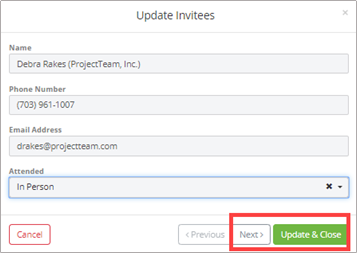The image depicts a user interface for updating invitees. The prominent section showcases the details of an invitee named Deborah Rakes, who is associated with Project Team Inc. Her phone number is listed as 703-961-1007, and her email address is rakes@projectteam.com. The invitation status indicates that she will attend the event in person.

The interface includes several interactive elements: 
- A red rectangle labeled "Cancel."
- Three additional rectangles: two white ones labeled "Previous" and "Next," and one green rectangle with the label "Update and Close" written in white.
- There is an additional red border surrounding both the "Next" and "Update and Close" buttons, highlighting their position and possibly their importance in the interface sequence.